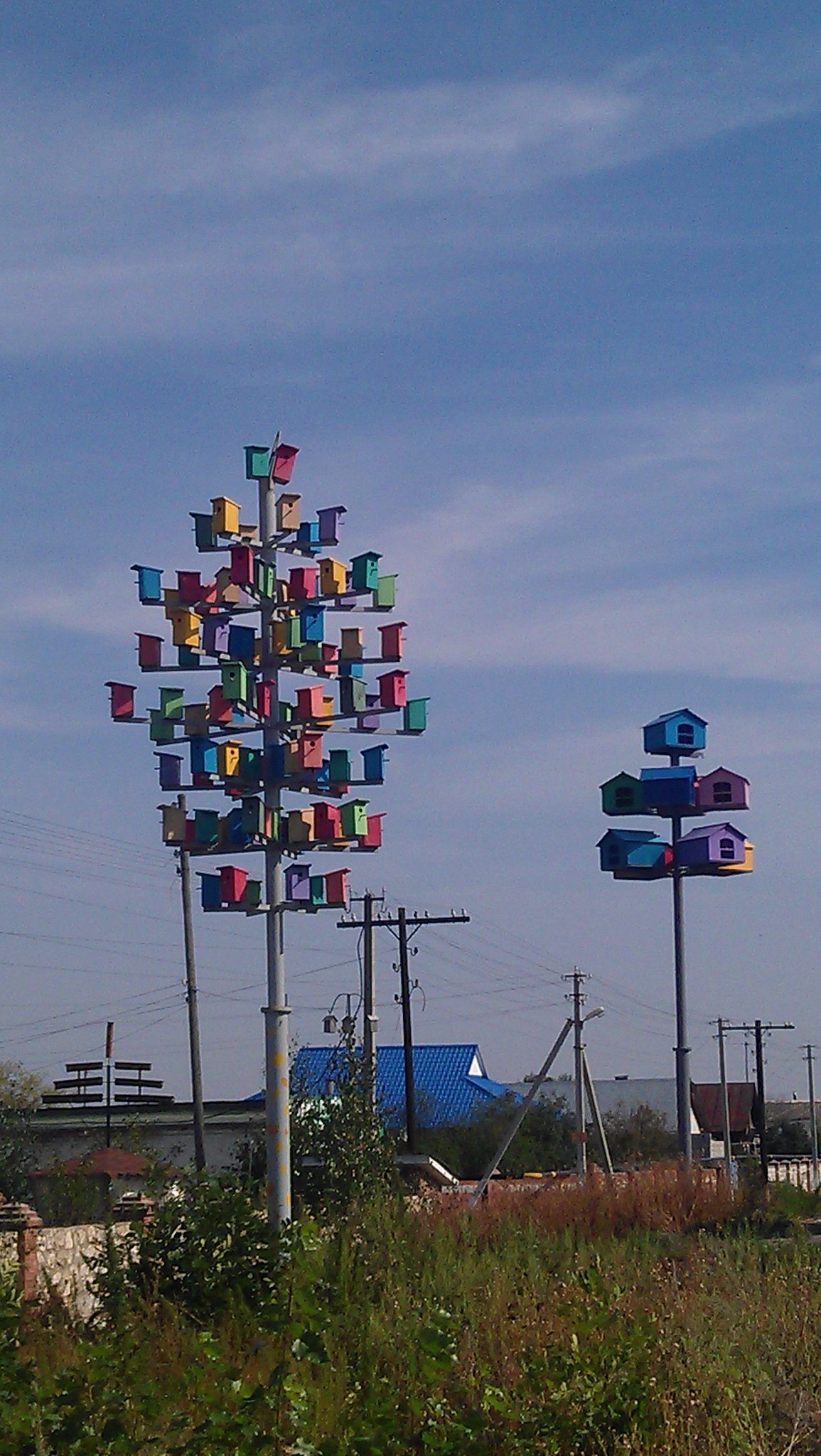This photograph captures an open field adorned with two central tall metal poles outfitted with numerous birdhouses. The pole in the foreground showcases a striking array of small, vibrant birdhouses, each painted in a solid color of the rainbow: yellow, orange, red, green, blue, and purple. These birdhouses are arranged in multiple tiers, vertically aligned in an intricate pattern resembling a whimsical village for birds.

In the background, the second pole features larger and wider birdhouses painted in an assortment of colors, including blue, purple, green, yellow, and red. These birdhouses appear more spacious, suggestive of miniature ranch-style homes, providing a varied contrast to the smaller structures in the foreground.

The surrounding landscape consists of a field with patches of grass and weeds growing sporadically. Beyond the field is a low retaining wall that likely borders a street, implied by the presence of telephone wires extending parallel to the road. In the distance, there are a few houses with roofs painted in shades of blue, gray, and brown, adding a touch of suburban life to the scene.

Above, the sky is predominantly blue with a scattering of light white clouds, providing a serene backdrop to this colorful and quaint arrangement.